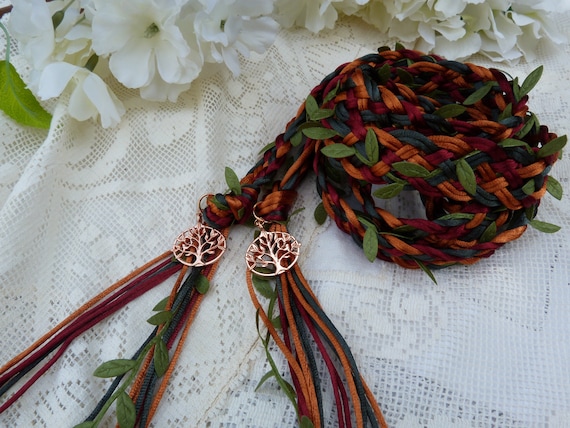The image showcases a close-up of a beautifully intricate macrame piece set against a lacy, beige tablecloth, creating a delicate and decorative appearance. The macrame features multiple colored strings, primarily in shades of red, orange, green, and dark gray, skillfully braided and twisted together. Interspersed within the braids are small, thin green leaves, adding a touch of natural elegance. Two metal ornaments resembling the Tree of Life, made of light bronze, dangle from the macrame, providing a symbolic and decorative touch. Surrounding the macrame, white flowers and more greenery hint at a celebratory atmosphere, possibly a wedding, as suggested by other decorations in the background. The entire composition evokes a sense of intricate craftsmanship and gentle festivity.